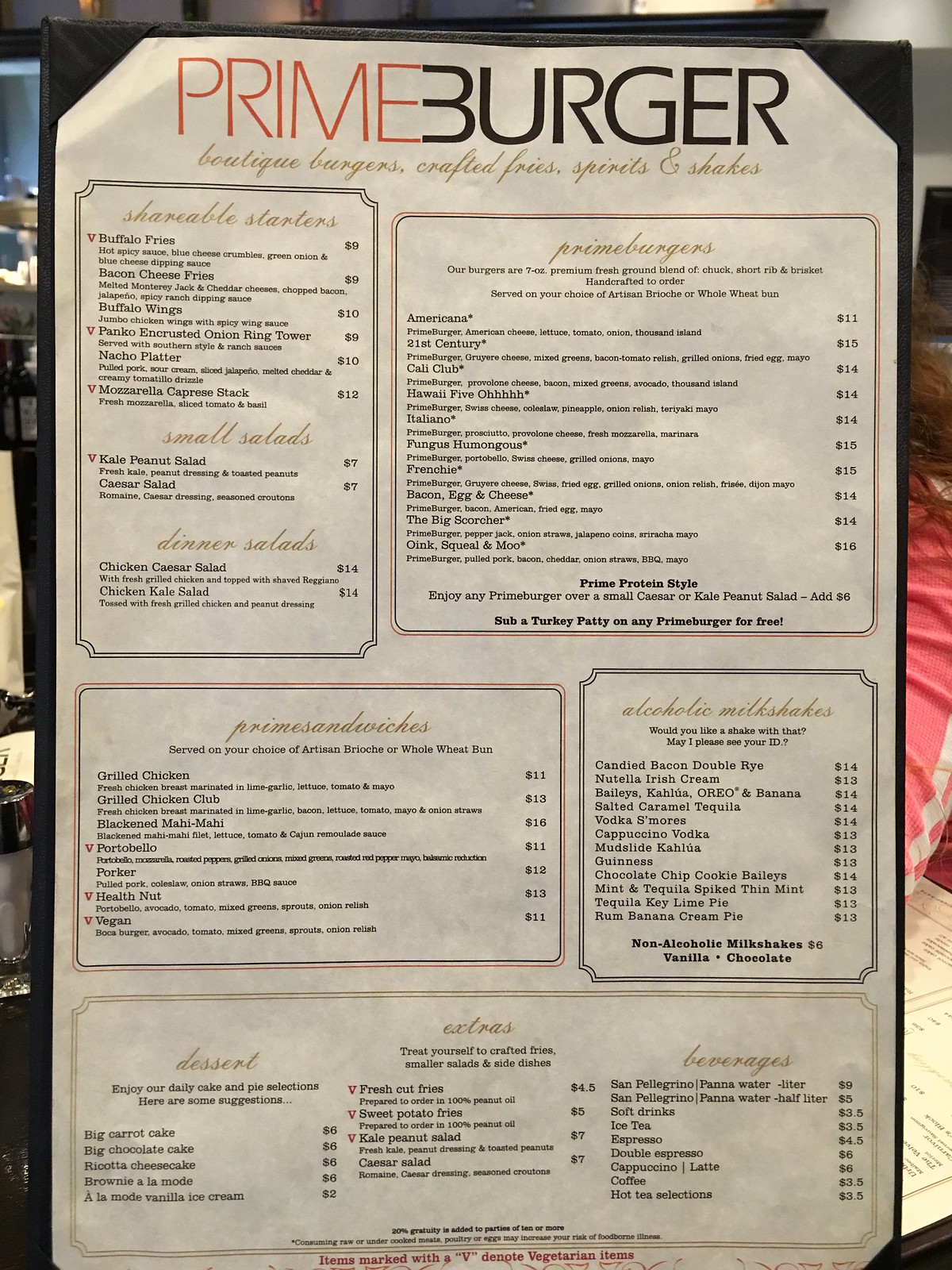This photograph, taken in a restaurant setting, prominently features a detailed menu as its central focus. The menu, titled "Prime Burger," is creatively designed with the letters "E" in "Prime" and "B" in "Burger" merging to form one giant letter each — a striking graphical element. "Prime" is written in red, while "Burger" is in black. Below the main title, in golden font, the text reads, "Boutique Burgers, Crafted Fries, Spirits & Shakes." 

The menu is divided into several sections, including "Shareable Starters," "Prime Burgers," "Alcoholic Milkshakes," "Desserts," and "Beverages." Each section lists various items with their prices, accompanied by brief descriptions in black font, highlighting the ingredients used.

The background reveals a cozy restaurant ambiance, with visible wine bottles on shelves and additional menus. A person with brown, wavy, curly hair wearing a pink long-sleeve sweater or shirt is partially visible on the right side of the image, seated at a table adorned with a salt shaker on the left. This meticulous layout and the detailed elements contribute to the inviting atmosphere captured in the photograph.